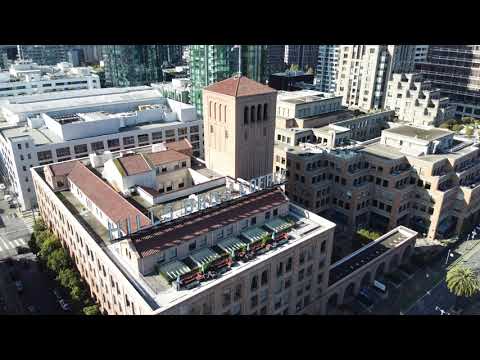This is a small, horizontal, rectangular image with a thick black bar at the top and bottom, framing a grainy, aerial photograph of a bustling urban area, likely captured by a drone. In the foreground, there's a three or four-story building, possibly condominiums or apartments, featuring a rooftop pool, cabana areas, and other rooftop structures. Adjacent to this building on the right, there’s a five or six-story building with the top two floors recessed, also likely serving as residences. The background is densely populated with taller buildings and skyscrapers, many of which are cut off at the top edge of the image, suggesting a busy, high-rise cityscape reminiscent of New York City. These buildings, primarily beige and white, are adorned with hundreds of windows, evidence of the congested, high-density urban environment. Streets weave beneath these buildings, with a significant shadow cast upon the street from a large, unseen skyscraper possibly to the left, indicating a vibrant and densely packed city atmosphere.